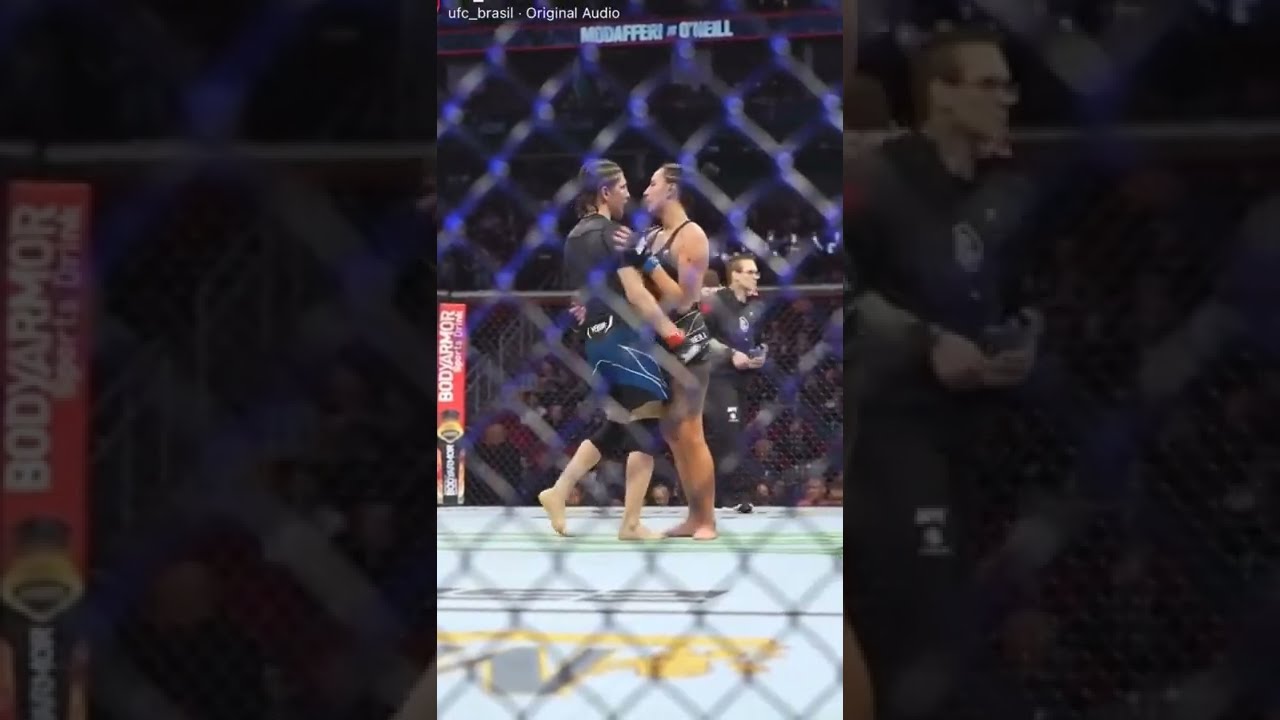The image depicts an intense moment in a UFC match, captured through the confines of a chain-link fence with blue lights accentuating its cross-sections. Centered in the action are two female fighters locked in a struggle. The fighter on the left, wearing a black short-sleeve shirt and blue pants with white stripes, is seemingly executing a kick, while the fighter on the right, dressed in a black tank top and grayish shorts, counters her move, suggesting a grappling scenario. Both have their hair tied back, possibly in braids or cornrows, adding to the fierce atmosphere.

The octagon's floor beneath them is a light blue with an indistinct green symbol partially visible, alongside some undecipherable black text and a potentially yellow star, contributing to the ambiance of the scene. In the background, a referee dressed in a blue shirt adorned with a central badge and long black pants stands attentively, although his arm's positioning appears to align oddly with the fighters, creating an illusion. Rows of an eager audience can vaguely be seen past the fighters, engrossed in the unfolding match.